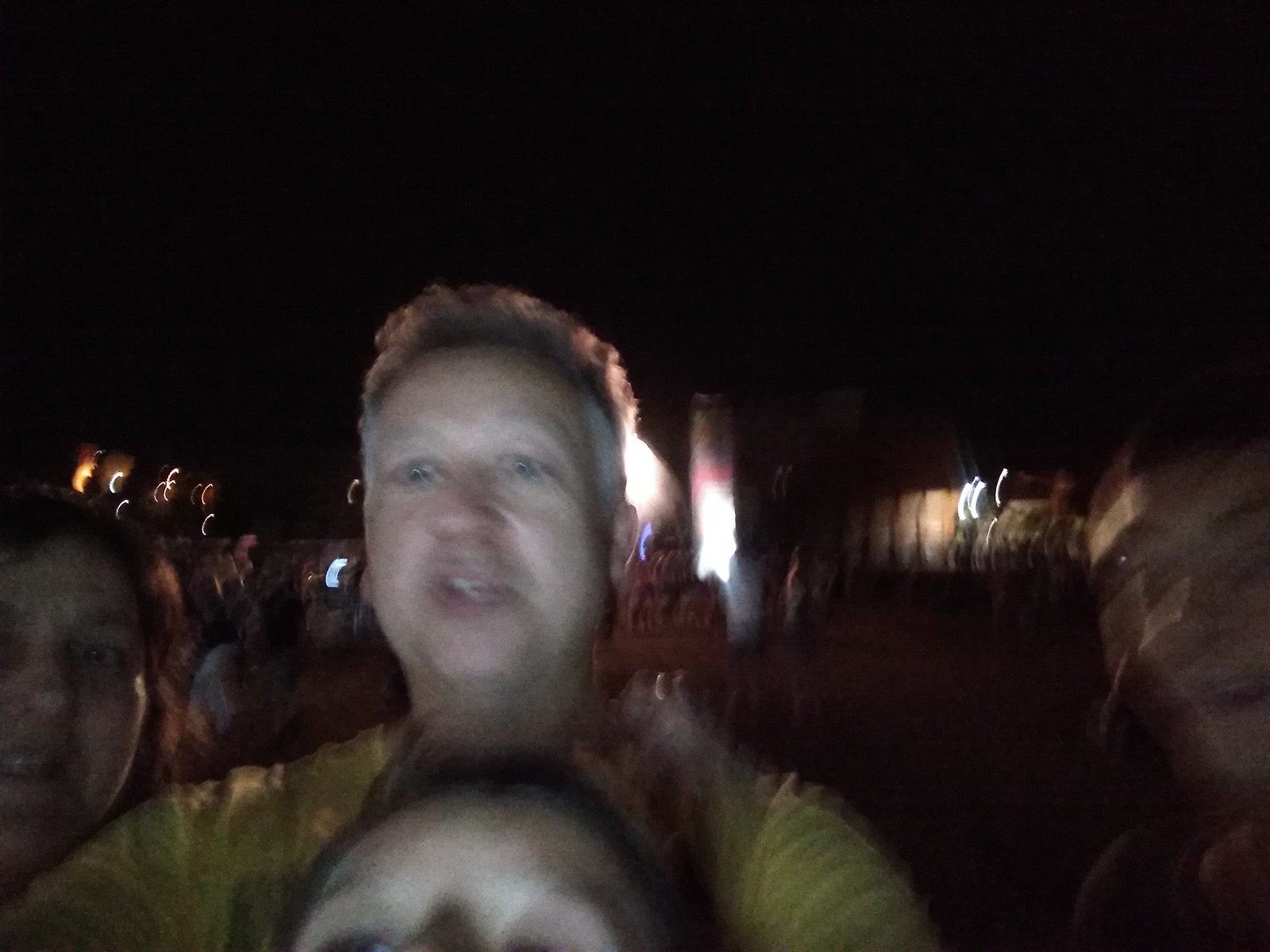A blurred nighttime selfie captures four people against a pitch-black sky dotted with indistinct building lights. Two individuals are positioned left of center, near the bottom of the frame: a Caucasian male with short, graying brown hair and blue eyes, clad in a yellow shirt, stands partially obscured. Directly in front of him, only the top of a shorter Caucasian person’s forehead with light brown hair is visible. To their left, a middle-aged Caucasian woman with long, dark brown hair stands out in the group. On the far right, another Caucasian male with short dark brown hair and brown eyes completes the scene, lending a sense of camaraderie to this unguarded, spontaneous moment.